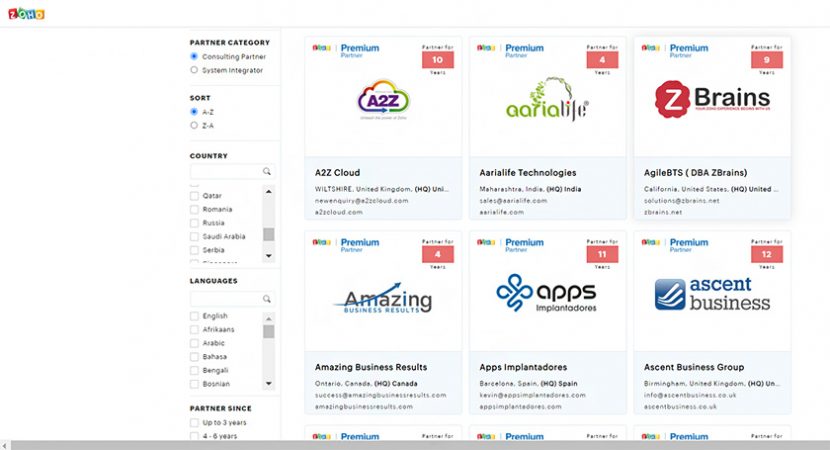The image captures a screenshot from a webpage designed for selecting consulting partners and system integrators. At the top of the page, partially obscured by a "Save" button, are the headings "Partner Category," "Consulting Partner," and "System Integrator." Users can sort these partners alphabetically from A to Z or Z to A. Below, there's a filter for countries, listing several options such as Romania, Russia, Saudi Arabia, and Serbia. Another dropdown menu allows users to select a language, starting with English and including various others. Under the heading "Partner Since," users can filter by duration options such as "up to three years" and "four to six years," though the list appears to be cut off.

The page features clickable rectangular areas arranged in a grid, with three items per row. The top row includes "A to Z" (using the numeral '2'), "Aeriolife," and "Zbrains." The bottom row displays "Amazing Business Results," "Apps," and "Ascent Business." Each rectangle likely offers more detailed information or directs the user to additional resources related to the respective partner or service.